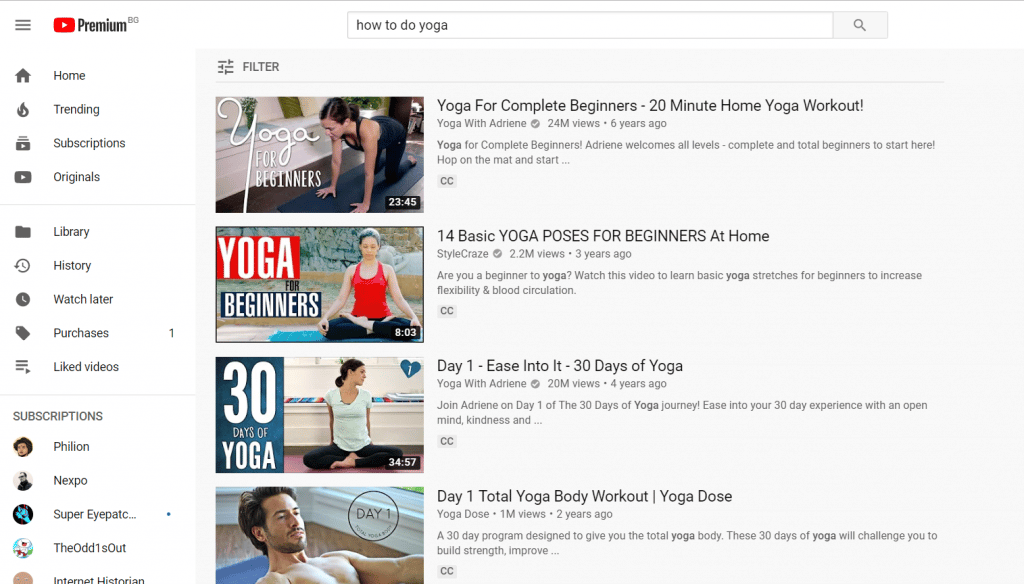In this image, we are looking at a YouTube webpage displaying results for a search query. At the top of the page, the YouTube logo is visible alongside a "Premium" badge. Below this header, a vertical navigation menu includes options such as Home, Trending, Subscriptions, Originals, Library, History, Watch Later, Purchases, and Liked Videos.

The search bar at the top contains the query "how to do yoga," and the screen is showing a series of four video results related to this search. Each video has a thumbnail featuring a person performing a yoga pose.

1. The first video is titled "Yoga For Complete Beginners - 20 Minute Home Yoga Workout" and has garnered 24 million views over six years.
2. The second video, titled "14 Basic Yoga Poses For Beginners At Home," has 2.2 million views and was uploaded three years ago.
3. The third video is named "Day 1 - Ease Into It - 30 Days of Yoga" and has received 20 million views in four years.
4. The fourth video is titled "Day 1 - Total Yoga Body Workout | Yoga Dose" and boasts 1 million views from two years ago.